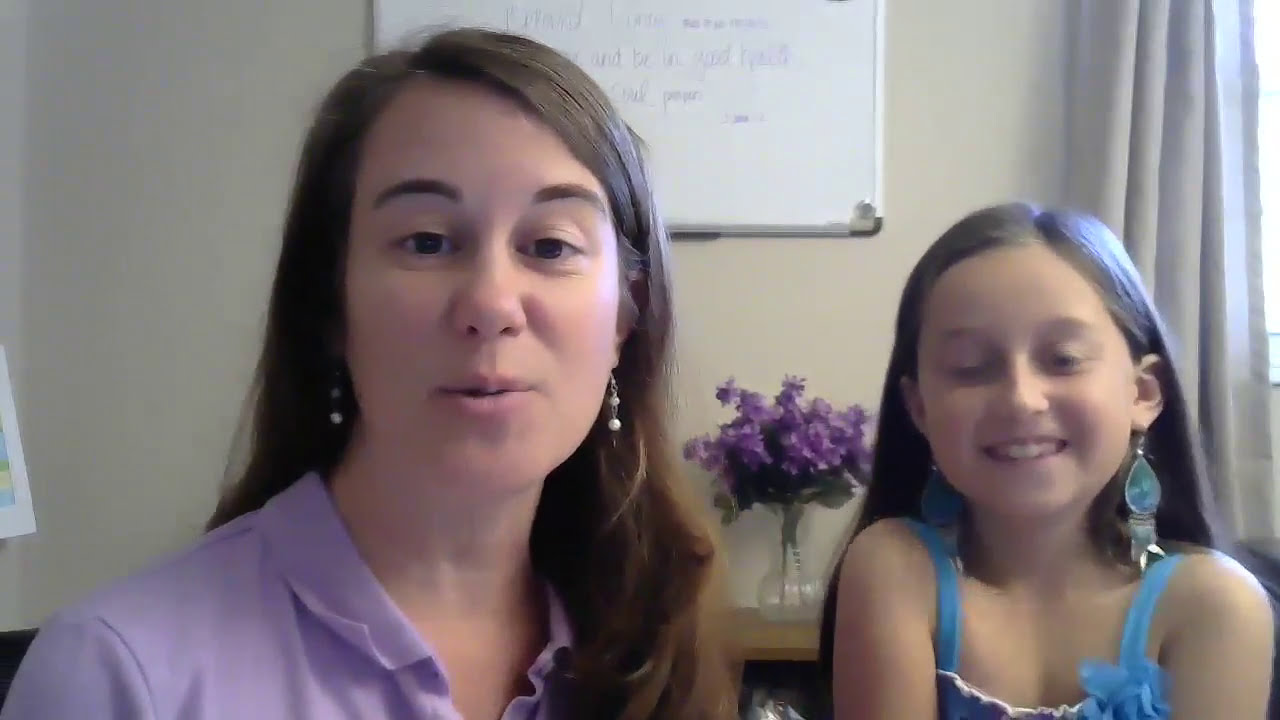In this image, an older woman and a young girl, possibly a mother and daughter, are seated in a room. The woman, who appears to be in her 30s, has long brown hair, is wearing earrings, and a purple or lilac-colored collared shirt. The young girl, likely around 9 or 10 years old, also has brown hair, turquoise earrings, and a blue dress with blue shoulder straps. The woman is speaking while the girl smiles with her eyes slightly closed. Behind them is a gray wall with a whiteboard that has purple writing on it, though the text is not clearly visible. A clear vase holding purple flowers with green leaves is situated on a brown wooden table behind them. To the right, there is a window with light gray or violet drapes, partially folded. Additionally, a paper board with blue, yellow, and green details can be seen in the background. Light streams in softly through the window, adding to the warm ambiance of the room.